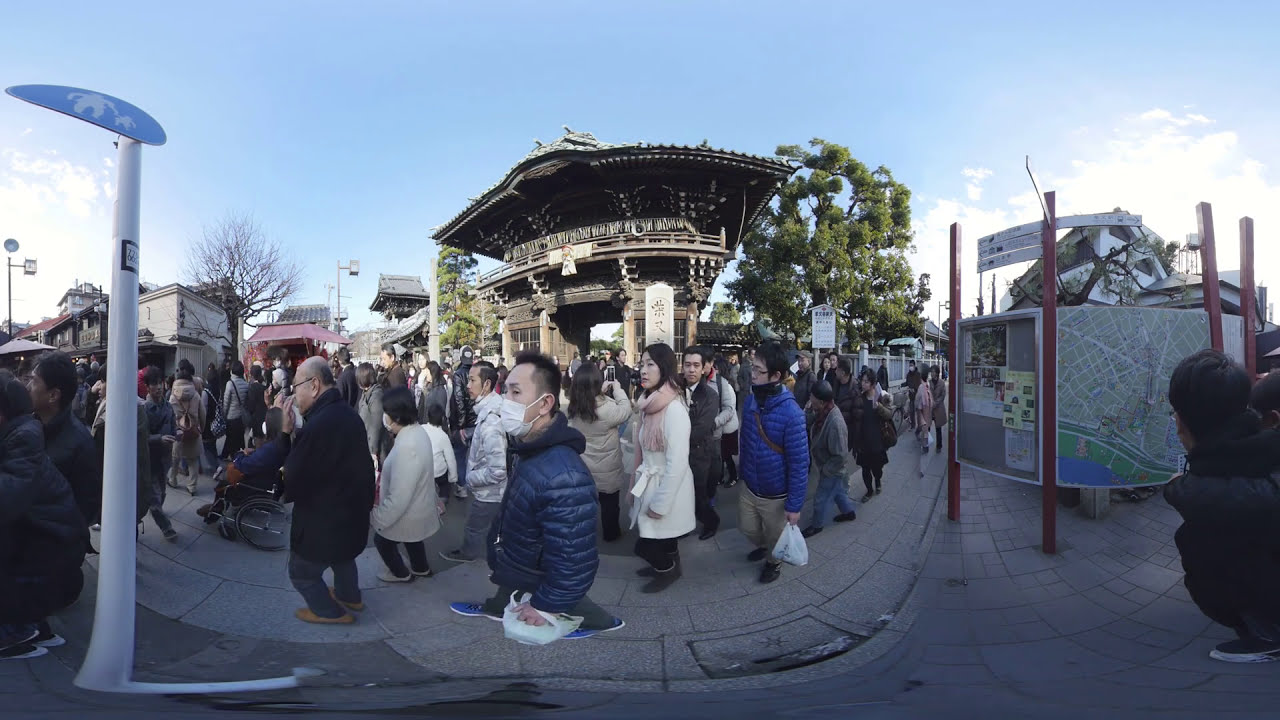The photo depicts a bustling street scene in Chinatown, featuring a large crowd of around 50 to 100 people walking towards the left on a concrete sidewalk. The crowd includes individuals wearing masks, blue and white coats, indicating it might be winter. In the middle of the background, there is a prominent, ancient Asian-style brown building or gate, surrounded by mostly leafless trees, suggesting a winter scene. On the street corner to the left, a white metal pole with a blue oval sign illustrating an adult holding a child's hand is visible. To the right, there are maps and directional guides on red metal poles, helping people navigate the area. The sky is bright with some white clouds, enhancing the vividness of the outdoor setting. Additional white square buildings are visible in the background, completing the urban landscape.